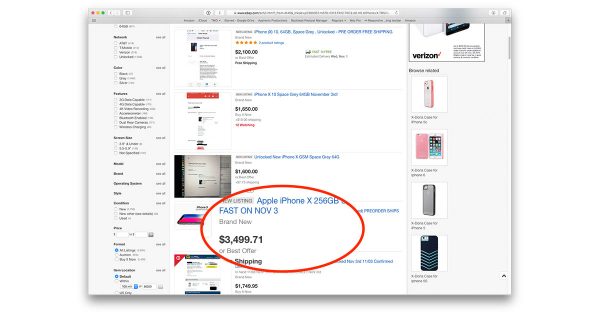**Descriptive Caption:**

The image features a small, detailed section of a website, likely an online marketplace, with various listings and navigation elements.

**Top of the Image:**
- Gray header running from left to right.
- Search bar prominently displayed, though illegible upon magnification.

**Left Side:**
- Column of selectable options in black text accompanied by checkboxes, but text is unreadable despite enlargement.

**Main Content Area:**
1. **First Listing:**
   - White background.
   - Item name in blue text, unreadable due to blurriness.
   - Five gold stars indicating ratings.
   - Text below stars possibly reading "52,100 UOD," followed by "plus shipping."
   - Item description and picture indistinguishable due to blurriness.

2. **Second Listing:**
   - Item name in blue text, illegible.
   - Possible price: "$2,000."
   - Another item name in blue, followed by a black price reading "1,650.00."
   - Red text underneath, unreadable.

3. **Third Listing:**
   - Blue text for item name, illegible.
   - Price in black, "3,499.71."
   - Gray banner stating "New Listing" in black letters.
   - Detailed description: "Apple iPhone X 256 GB," marked with a red oval. Mention of "fast on November 3," "Brand New," and an option of "or best offer."
   - Indication of "free shipping."
   - Additional blue text, unreadable.

**Bottom Right Content:**
- Visuals of multiple cell phones:
   - Four small pictures: a pink and white cell phone, a purely pink cell phone, a gray cell phone, and a black case with blue stripes.
   - App icons on phone screens present but text unreadable.

**Overall:**
The layout suggests a busy online marketplace with various listings, descriptions, and pricing details. Despite the general blur, it is clear that smartphones are prominently featured, particularly the Apple iPhone X 256 GB with extensive details and markings highlighting its listing.